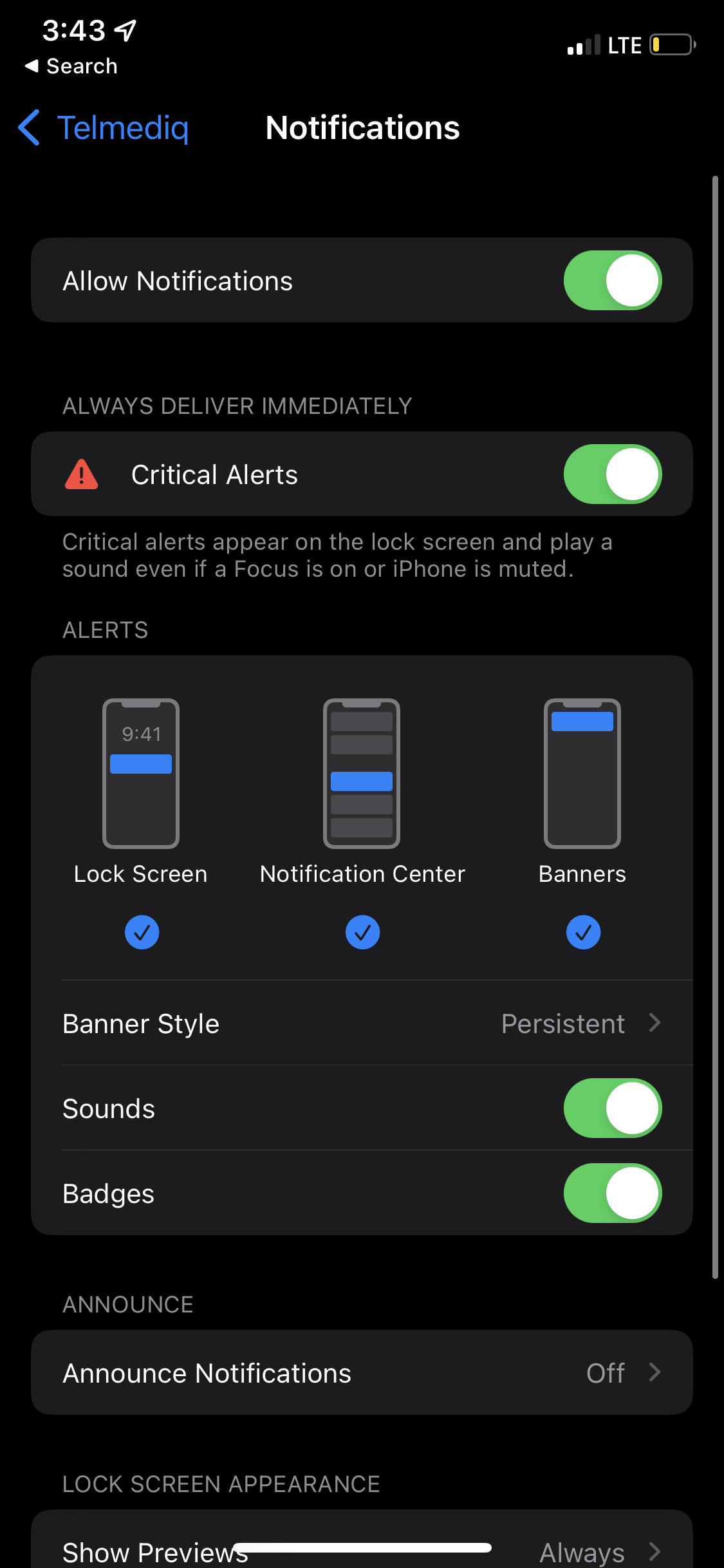A meticulously captured screenshot from an iPhone, showcasing the Notifications settings. The screen, displaying the current time as 3:43, indicates that the user is actively allowing notifications and has enabled critical alerts to be delivered immediately. Visible are the options for Lock Screen, Notification Center, and Banners, all of which are enabled to produce sounds and display badges upon receiving notifications. The device, connected to the LTE network, hints at a possibly Irish service provider. The user’s battery icon is yellow, signifying that the Battery Saver mode is activated. Notably, the Announce Notifications feature has been turned off, while the notification alerts for the Lock Screen, Notification Center, and Banners remain active. The selected banner style is Persistent, ensuring that they are continually visible until actioned. Additionally, message previews are always displayed on the lock screen.